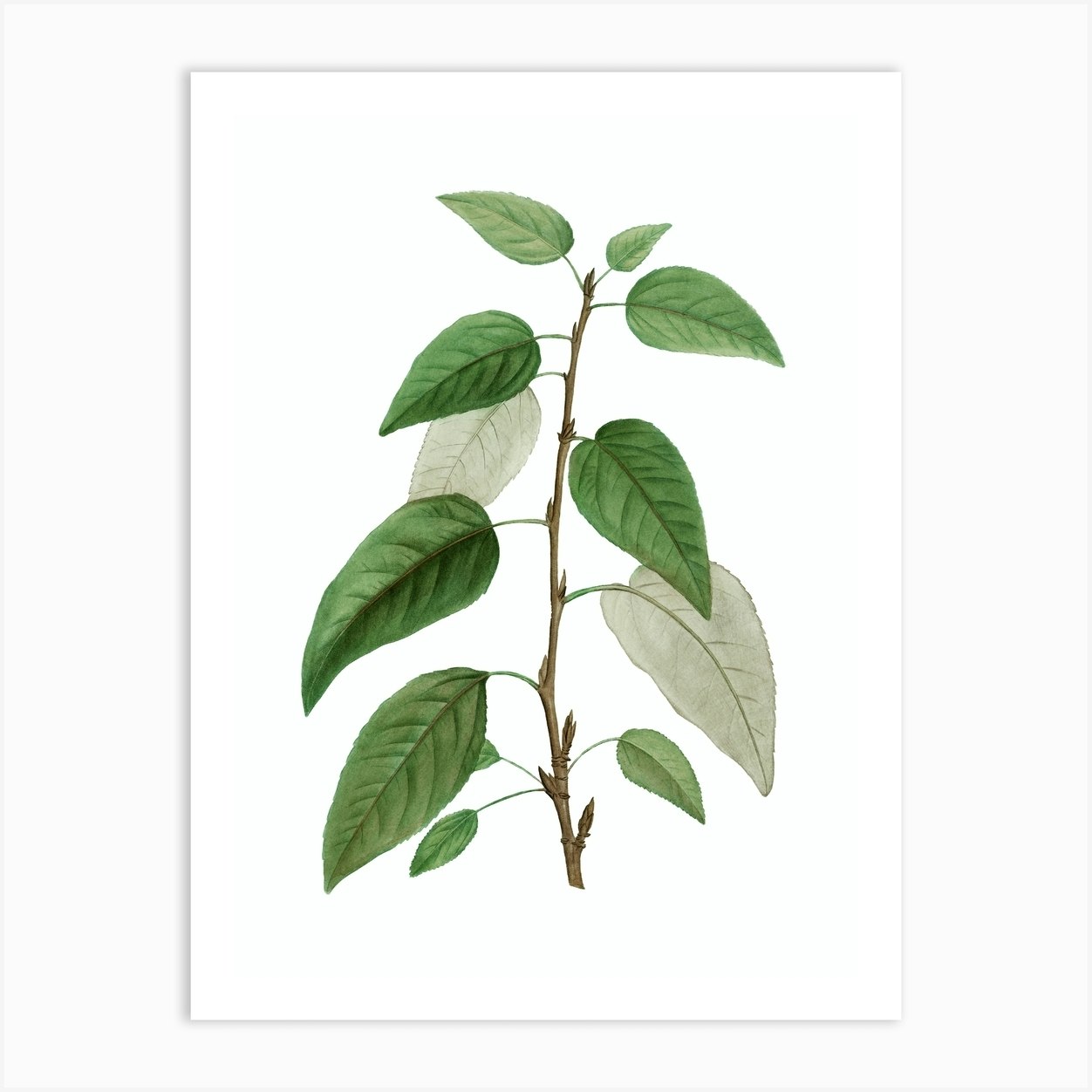The image depicts a detailed illustration of a plant against a white or light gray background, resembling a scanned piece of paper. The central feature is a thin, brown stem that extends vertically. This stem is adorned with various leaves arranged symmetrically on either side. The leaves vary in size, with smaller, teardrop-shaped leaves at the bottom, and larger ones as you move upward. On the left side of the stem are four prominent green leaves, with one slightly lighter green leaf positioned in the background. On the right side, there are three large green leaves, also with a lighter leaf behind them. The leaves exhibit visible veins, enhancing their realistic appearance. There are small leaves at both the top and bottom on the right side, and the plant's structure reveals multiple nodes along the stem, possibly indicating where flowers might eventually form.